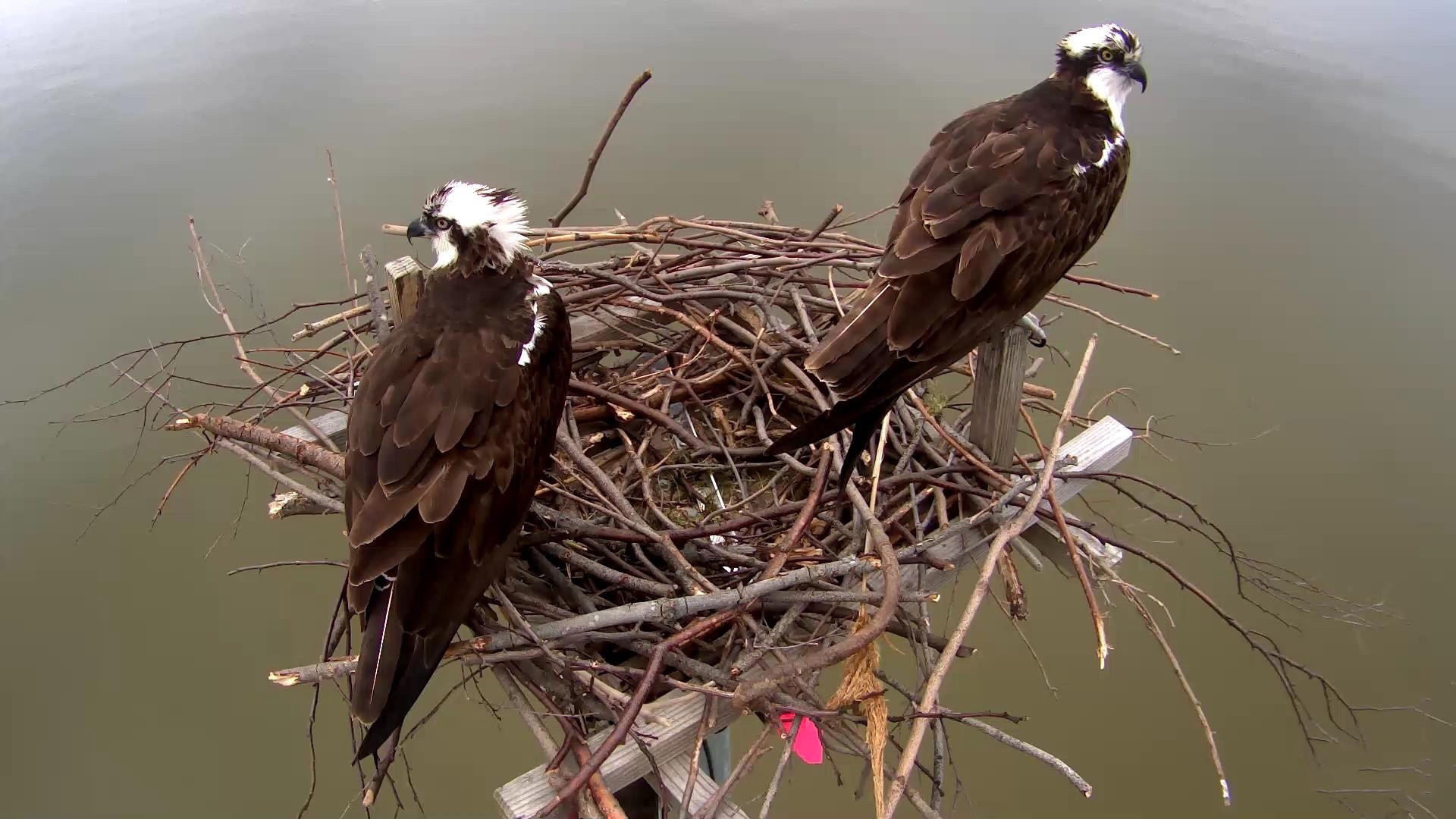This detailed photograph captures a close-up, top-down view of a pair of medium-sized raptors, likely a type of eagle or hawk, perched in their nest. The birds are adorned with predominantly brown feathers covering their bodies and wings, while the tops of their heads and necks exhibit patches of white, interspersed with brown around their eyes. Their sharp, curved beaks are distinctly black.

Positioned in a nest constructed haphazardly from various sticks, the raptors are seen atop a wooden platform designed for nesting, suggesting human intervention in its construction. This platform stands above a body of still, greenish water, possibly indicating a lake or a swampy area. The birds' postures are noteworthy: one on the left faces straight ahead with its head turned left, and the other on the right has its body turned slightly right with its head tilted down and to the right. The serene setting and intricate details of the nest and birds highlight the natural elegance of the scene.